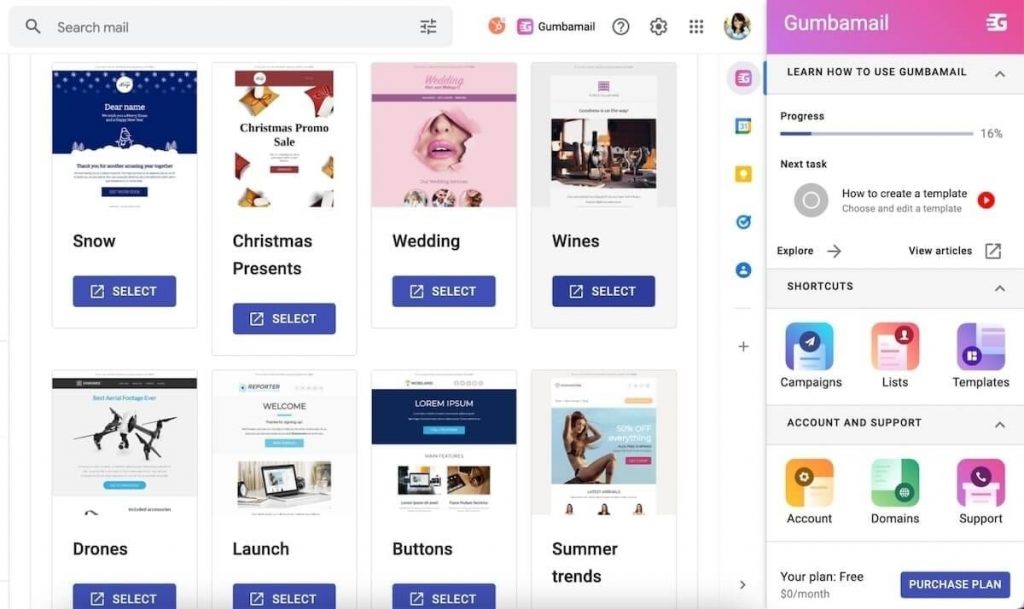This screenshot depicts the interface of Gumba Mail, an email service. At the upper left corner, there is a search box with the placeholder text "search mail" displayed in light gray. Adjacent to this, on the right, is a dropdown menu for selecting specific filters to refine search results. Further to the right, there is an orange icon followed by the Gumba Mail logo.

Continuing to the right, there is a circular help icon marked with a question mark, providing users with assistance when clicked. Next, a gear icon is present for accessing the settings menu. Adjacent to the settings icon is a grid of nine dots, presumably offering additional options within the service. 

To the far right, a small circular avatar appears, likely representing the user’s account; it features a cartoonish image of a woman. Below this top navigation bar, there are eight selectable boxes, each corresponding to different categories: snow, Christmas presents, wedding, wines, drones, launch, buttons, and summer, arranged in two rows.